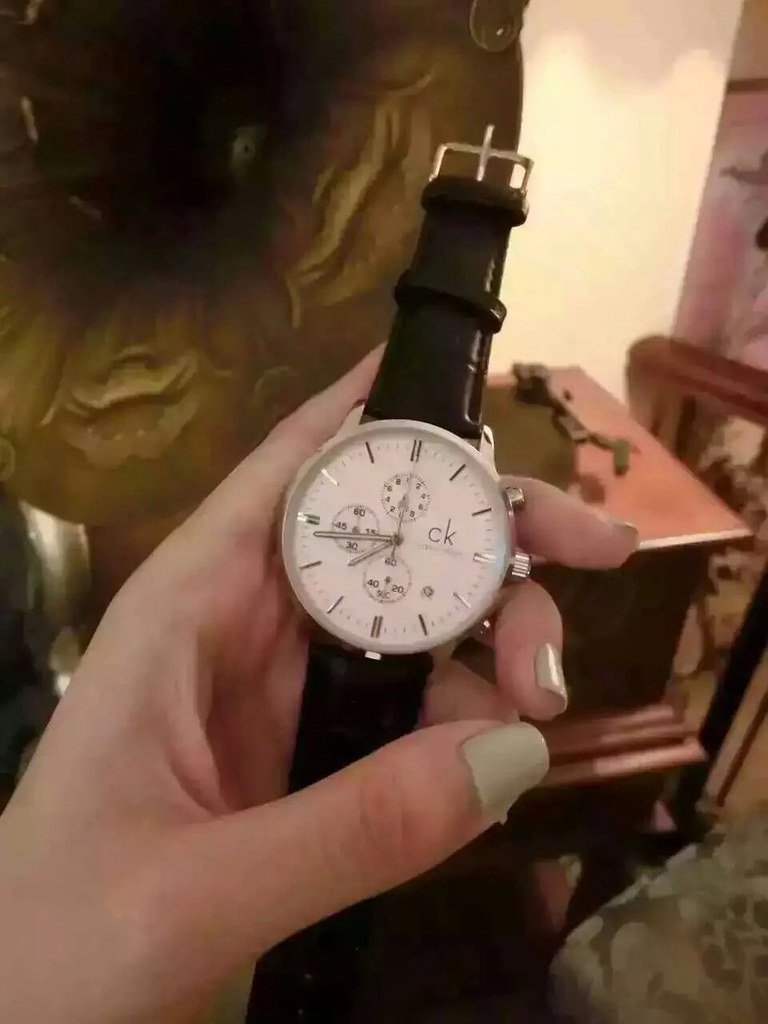This vertical photograph captures an elegant moment centered around a woman's left hand, delicately holding a sophisticated watch. Her thumb is positioned in the forefront, while her fingers eloquently frame the timepiece, securing it between her index, middle, and ring fingers. This luxurious dress watch boasts a black leather band, a pristine white face enclosed by a silver rim, and features three sub-dials within the main face. The prestigious branding 'CK' cleverly hints at the watch’s high-end status.

The background presents a rich tapestry of textures and elements with a distinct Victorian influence. Among these, an antique gramophone with its distinctive horn stands out, reminiscent of a bygone era. Adjacent to it, an ornate piece of antique furniture adds to the timeless ambiance, adorned in a palette of brass, brown, yellow, and olive green hues. The woman's fingernails are painted a muted, light olive green, complementing the color scheme and adding an additional refined touch to the composition.